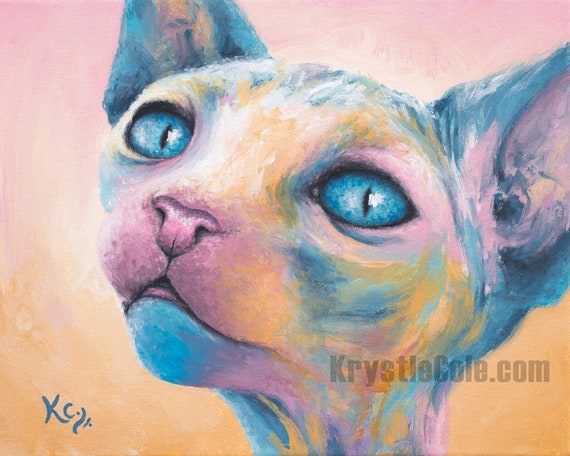The image features a headshot of a Sphinx cat, vividly depicted in a range of pastel colors including teal, blue, orange, pink, and yellow. The cat has striking teal-blue eyes with black pupils, framed by black outlines, and is positioned with its ears erect, looking slightly upward and to the left. The cat’s nose is pink, its cheeks blend between blue and yellow, and its bottom mouth and chin are blue. The artist has skillfully used a mix of colors for the cat’s skin, featuring shades of blue, white, green, and yellow on its forehead, while inside of the ears is painted pink. The background transitions from pink at the top to orange and then yellow at the bottom, enhancing the overall vibrant atmosphere. Despite its bright palette, the image conveys a slightly eerie feeling due to the depiction of the hairless cat. The artist’s initials, “KC,” appear in blue at the bottom left corner, while a watermark reading “crystalcoal.com” is located on the bottom right.